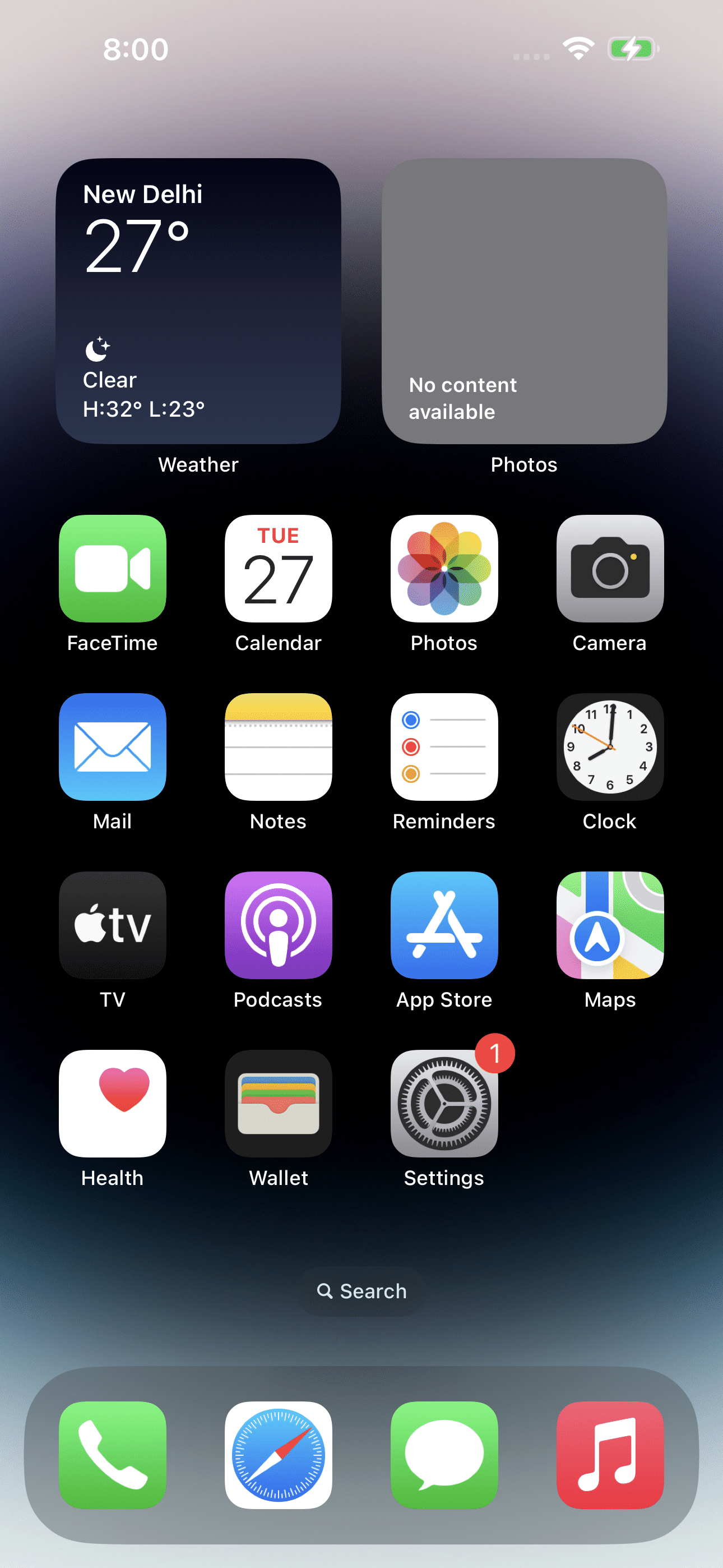A detailed screenshot of a smartphone's home screen.

At the top of the screen is a dark gray status bar. On the left-hand side, in white text, it displays the time as "8:00," without specifying AM or PM, suggesting it might be in military time. On the right-hand side, there is a Wi-Fi symbol indicating full signal strength, followed by a battery icon that is fully charged and features a white lightning bolt, indicating the phone is being charged.

Below the status bar, on the left side, there is a black square featuring bold white text that reads "New Delhi." Accompanied by a temperature reading of "27°," which could be in either Fahrenheit or Celsius. An icon depicting a moon and stars indicates clear nighttime weather. The high and low temperatures are displayed as "H: 32°" and "L: 23°."

Adjacent to this, toward the right, is a dark gray square with white text that reads "No content available" in the lower left corner. On this screen, "Weather" appears underneath on the left, and "Photos" on the right. Numerous app icons are displayed below.

From left to right, the visible app icons include:
1. **FaceTime** - A video camera icon on a teal background.
2. **Calendar** - A red "Tuesday" above "27" in black on a white calendar icon.
3. **Photos** - A multicolored pinwheel icon.
4. **Camera** - A camera icon on a gray background.
5. **Mail** - A white envelope icon on a dark blue background.
6. **Notes** - A notebook paper icon with an orange band at the top.
7. **Reminders** - A white icon with three lines and circles in blue, red, and orange, along with a zero.
8. **Clock** - A clock icon.
9. **TV** - A black square with the Apple logo and the word "TV".
10. **Podcasts** - A purple icon with concentric white circles resembling an exclamation mark.
11. **App Store** - A dark blue icon with an "A" made of sticks.
12. **Maps** - An icon with a blue circle, a white arrow, and a red outline.
13. **Health** - A white circle with a red heart in the top right corner.
14. **Wallet** - A gray wallet icon with bands of blue, orange, and green.
15. **Settings** - Two black gears on a light gray background with a red circle and the number 1.
16. **Search** - A magnifying glass icon.
17. **Phone** - A dark green background with a phone symbol.
18. **Siri** - A white background with a blue compass-like icon featuring a red point.
19. **Messenger** - A dark green icon with a white speech bubble.
20. **iTunes** - A red icon with a white musical note.

This comprehensive description captures the details of the smartphone's home screen, highlighting both the status bar and each individual app icon present.